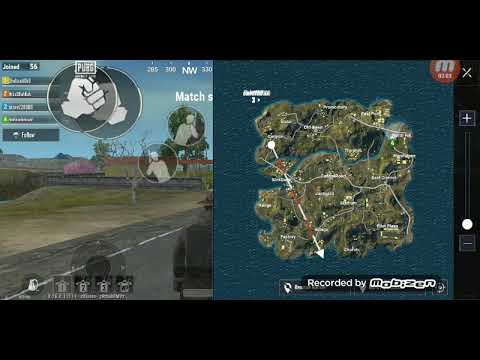This image appears to be a screenshot from video game gameplay, featuring a split-screen layout with a black background. The left side showcases a third-person perspective of a character dressed in a long black jacket and possibly wearing a cowboy hat, walking or standing on a paved road flanked by trees and branches. Above the character, an emblem of a fist is visible. Alongside the character, there are clickable elements, likely for changing weapons, indicating that it might be a shooter game. Partial text that includes "NW" and the word "match" is also visible.

On the right side of the screen, there's an overhead view of a piece of land resembling an island, surrounded by dark water. This section of the image includes a map with arrows, aiding navigation. The map display partially covers the gameplay on the left side, potentially indicating that the game is paused while the map is consulted. There is a watermark at the bottom right corner that reads "Recorded by Mobizen," though the remaining text is too small to discern. The color palette includes black, white, gray, silver, red, orange, pink, green, and various shades of brown.